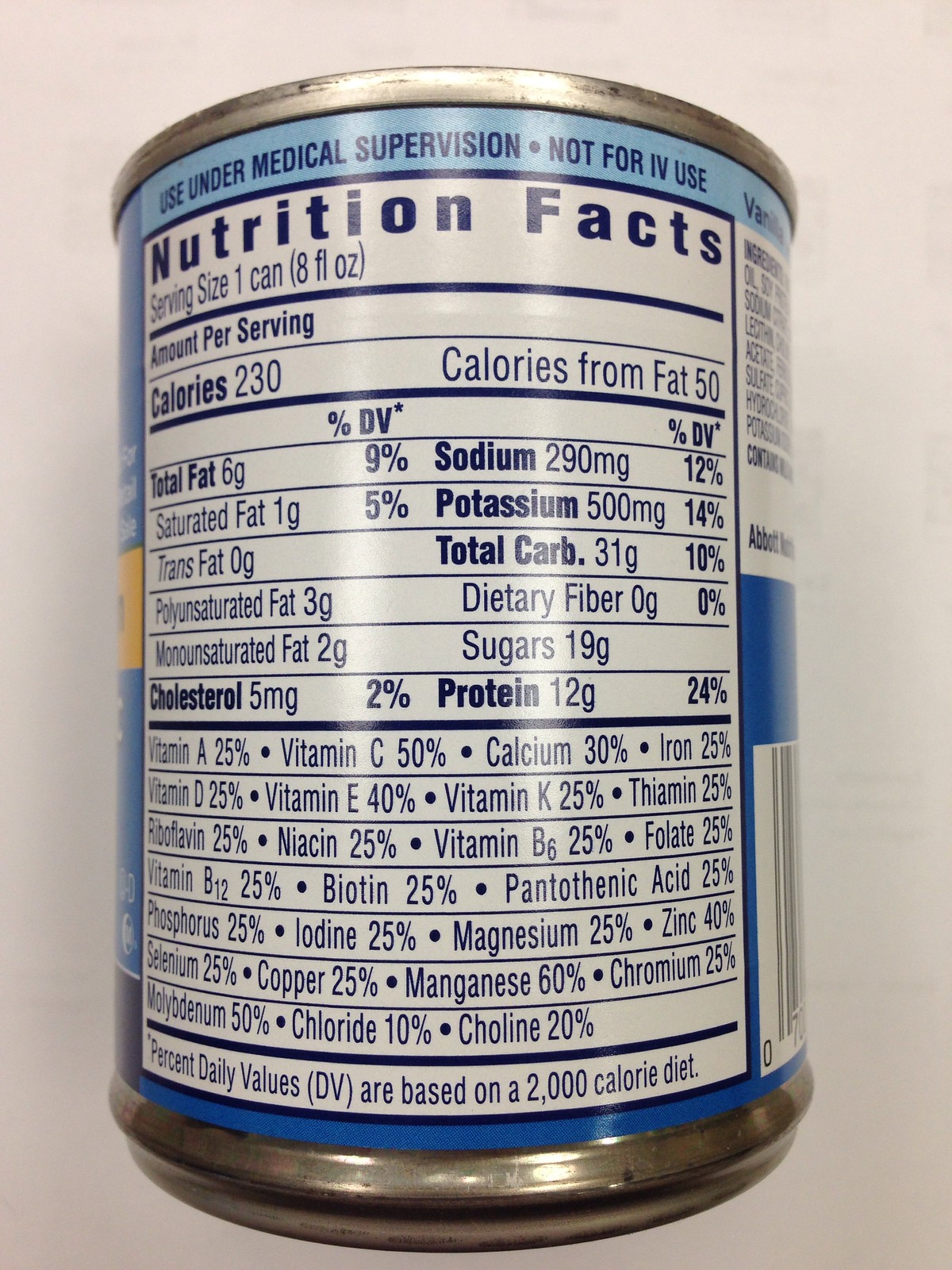Detailed Caption:

This image displays the back of a silver can containing a food-related product, presumably designed for individuals with specific dietary needs or medical conditions. The label is predominantly blue and white with clearly legible black text. The label provides extensive nutritional information, including a serving size of one can (8 fluid ounces). It explicitly states that the product should be used under medical supervision and is not intended for intravenous use, emphasizing the importance of proper administration. The nutritional values are detailed and are based on a standard 2000 calorie diet, ensuring consumers are well-informed about their dietary intake.